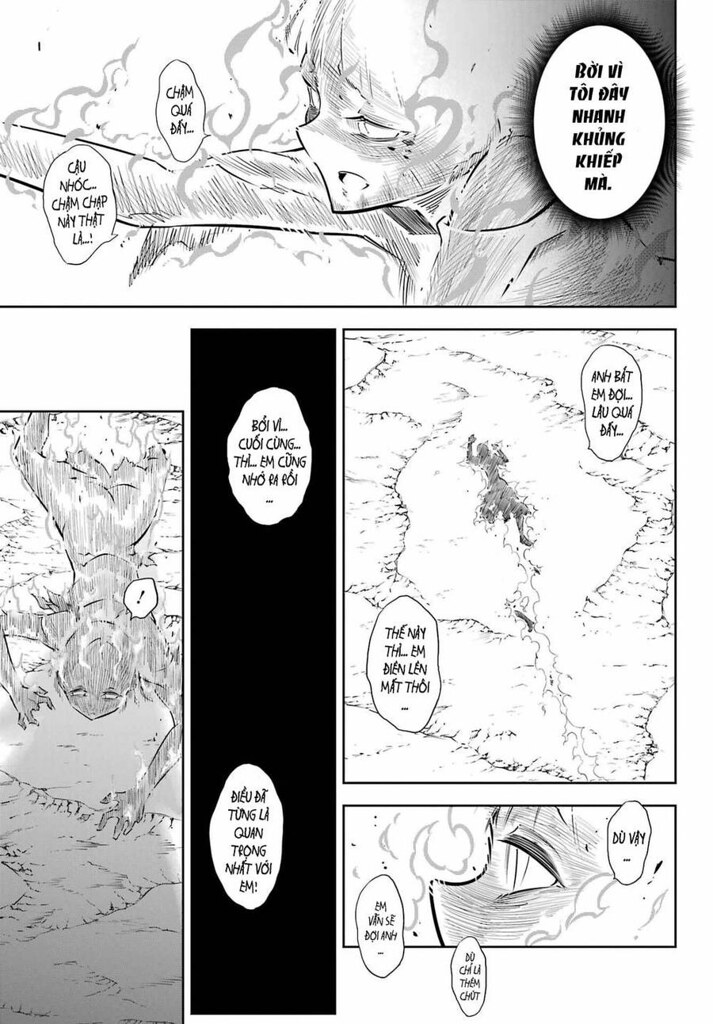This detailed image showcases a multi-paneled cartoon, likely rendered in shades of black, white, and gray, with text in what appears to be Vietnamese or another Southeast Asian language. The cartoon features four different characters and includes various scenes. One panel depicts an individual crawling on the ground, possibly in the presence of a monster or some other looming threat. Another panel highlights a close-up drawing focused on the eye and nose of a character, evoking a sense of surprise or fear, without showing the entire face. Additionally, there are panels that illustrate individuals swimming, possibly in a lagoon. The overall style of the cartoon is consistent throughout, with detailed text accompanying the drawings in each panel to convey the narrative.